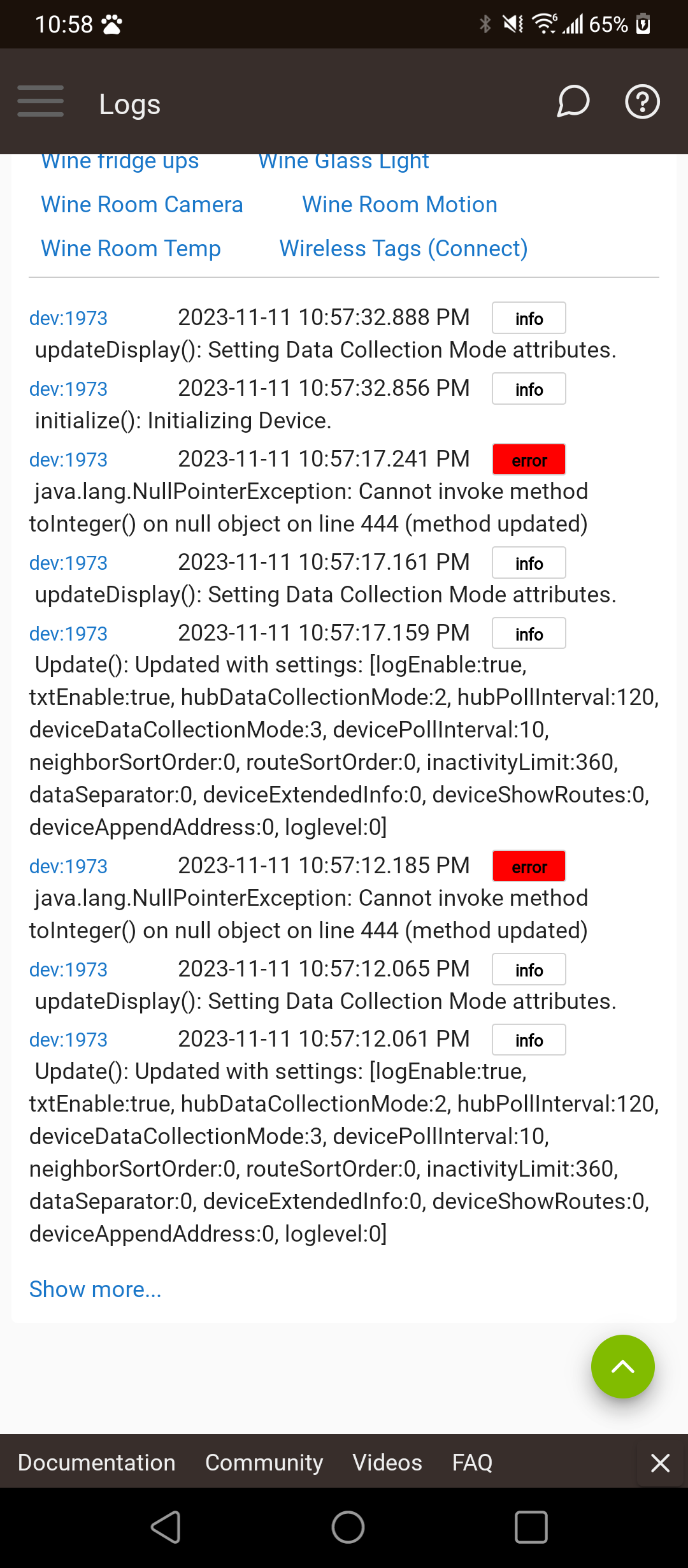The screenshot displays a log on a smartphone. In the top right-hand corner, there is a timestamp showing 10:58, along with a battery life indicator at 65% and an icon indicating that the sound is off. These elements are positioned within a black band at the top of the screen.

Just below, a dark gray band appears. On the left side of this band are three gray horizontal lines, followed by the word "Logs" written in white. Over on the right side of the band, there is a conversation icon and a white circle with a question mark inside.

Below this band, blue text lists several items: "Wine fridge ups," "Wine glass light," "Wine room camera," "Wine room motion," "Wine room temp," and "Wireless tags," with "connect" in parentheses.

The main body of the screenshot contains multiple lines of code. Each section starts with blue text stating "DEV: 1973," followed by lines of text beginning with the date "2023-11-11” and a timestamp. To the right of each timestamp is a rectangle labeled "info." Some code sections also feature a red box with the word "ERROR" written inside it.